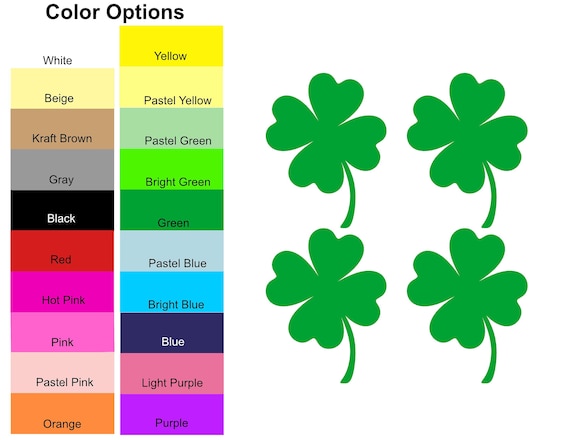The image features a detailed color palette against a white background, often found in hardware stores like Lowe's or Ace Hardware, for selecting paint colors. The palette on the left is arranged in two columns and includes a spectrum of colors: white, beige, craft brown, gray, black, red, hot pink, pink, pastel pink, orange, yellow, pastel yellow, pastel green, bright green, green, pastel blue, bright blue, blue, light purple, and purple. Each color is presented within a square labeled with white text. On the right side of the image, there are four green four-leaf clovers, evenly spaced in a row—two on the top and two on the bottom. The clovers, complete with heart-shaped leaves and small stems, are placed to possibly complement the green shades on the color chart, adding a thematic element to the image.